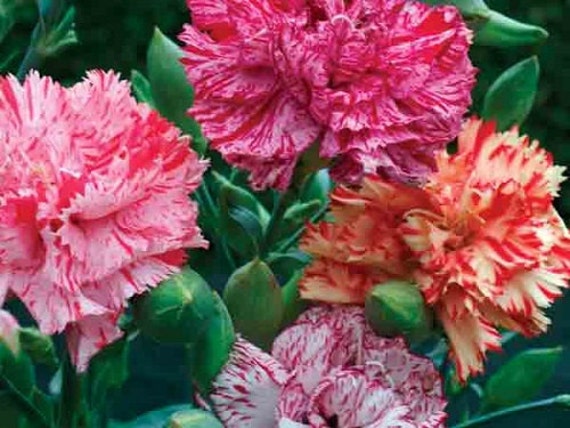This vibrant and detailed image captures a photorealistic close-up of chrysanthemum flowers in full bloom. Dominating the scene are four distinct flowers amid a lush backdrop of bright green leaves and green stems. At the top, a flower showcases a striking blend of reddish and pink hues. On the left, another flower displays mostly pink petals with delicate light red accents. To the right, a flower stands out with its yellowish petals accented with red marks. Finally, at the bottom, there is a predominantly white flower graced with subtle pink parts. The flowers appear upright and firmly rooted in the ground, and though the photograph does not focus on any single flower completely, it offers glimpses from various angles, capturing their vibrant colors and intricate details amidst the greenery. The background appears slightly grainy, emphasizing the upfront beauty of this simple, yet elegant floral arrangement.